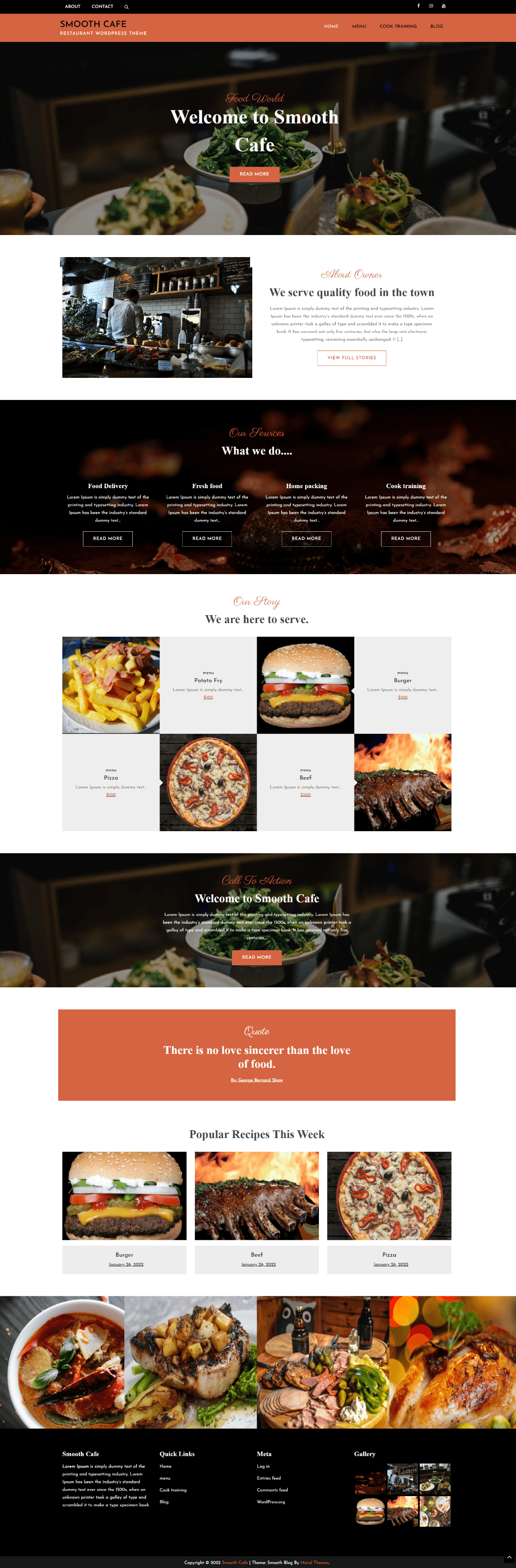Screenshot of Smooth Cafe's website:

At the very top of the website, the header stands out with an orange background. On the left side of this header, the site's name "Smooth Cafe" is prominently displayed. On the opposite side, the right side, there are four categories to navigate the site.

Just below the header, there is a central image that showcases an assortment of food on a plate, with the text "Welcome to Smooth Cafe" prominently displayed in the center. Beneath this welcoming message is an orange button.

Scrolling down, the next section features a photograph of a kitchen accompanied by some text on its right side. Below this, there's a long image labeled "What We Do" at the top, followed by eight blocks divided into four images and four text blocks. The images in this section depict a variety of foods: French fries, pizza, a hamburger, and what appears to be ribs, with each image center-aligned in its respective box.

Further down is another long banner-like image featuring a bowl of salad with text overlay. This section includes a header in the center, additional text below, and an orange button.

Continuing, there's an orange box with white text centered within it, followed by a section titled "Popular recipes this week." Below this title are three photographs showcasing popular food items: a hamburger, ribs, and a pizza placed from left to right. Each image has associated text beneath it.

Finally, at the bottom of the page in the footer, there are four images of different food types arranged horizontally from left to right. The footer also includes a body of text and several more images, completing the detailed presentation of the Smooth Cafe's website.